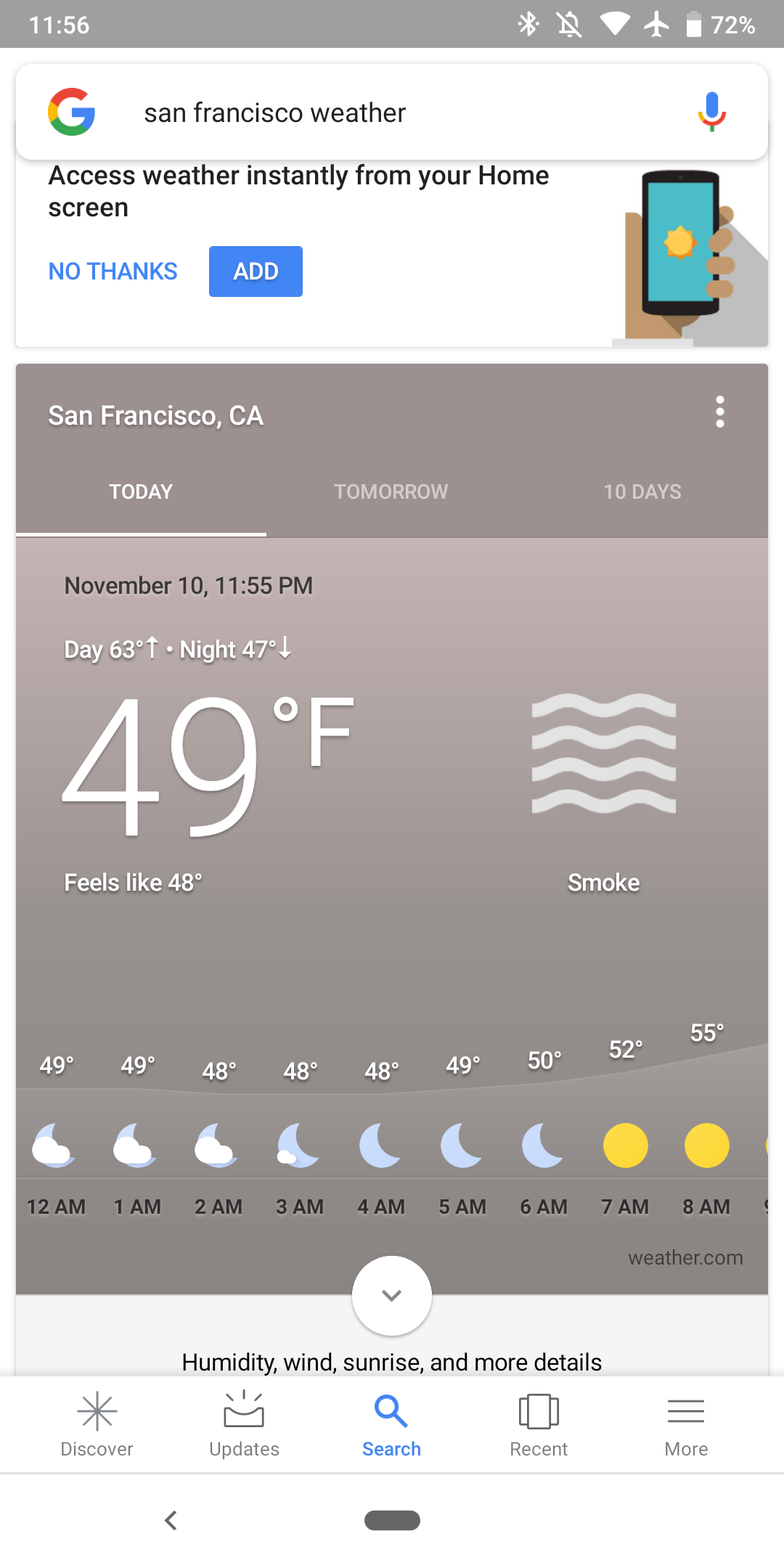The image shows a smartphone displaying the Google weather forecast for San Francisco. The top of the screen reads "San Francisco Weather," with a prompt beneath it suggesting users can instantly access weather updates from their home screen. There is an option for "No Thanks" on the left side and an illustration of a hand holding a phone with a sun icon on the screen to the right.

The interface consists of a darker beige top banner with options for viewing today's weather, tomorrow's forecast, or a 10-day outlook. The section focused on today’s weather is selected, showing details for November 10th at 11:55 PM. The current temperature is 49°F with a "feels like" temperature indicator, noting the conditions are smoky.

Beneath this, there's a timeline of hourly forecasts starting from midnight, displaying conditions like "mainly cloudy" alongside symbols such as the moon. Temperature readings are provided above each hourly forecast.

Further details include a section for humidity, wind, sunrise, and additional information, which can be expanded via a dropdown menu.

At the bottom of the screen, there is a navigation bar with options including Discover, Update, Search, Recent, and More; the Search option is currently highlighted in blue.